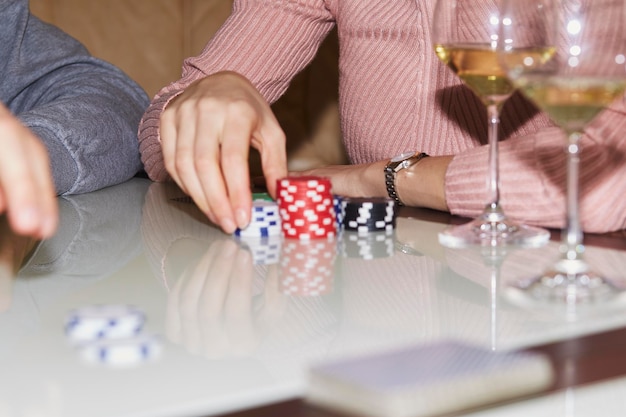In this image, a white table serves as the setting for a poker game, where only the torsos and arms of two individuals are visible. One individual is clad in a white and red striped shirt and has three stacks of poker chips in front of him: a tall stack of red chips, alongside smaller stacks of white and black chips. The other individual is wearing a light pink long-sleeved sweater and is reaching for a stack of white-and-blue poker chips. Both individuals have fair skin, and the person in the pink sweater has a watch on their wrist. The table features reflections of the people's arms and hands, adding depth to the scene. Flanking the players are two wine glasses filled with a chilled, pale yellow liquid, hinting at a relaxed atmosphere. In the blurred foreground, there's a deck of cards. This image is bordered, emphasizing the central activity while softly framing peripheral objects like the poker chips and drinks.